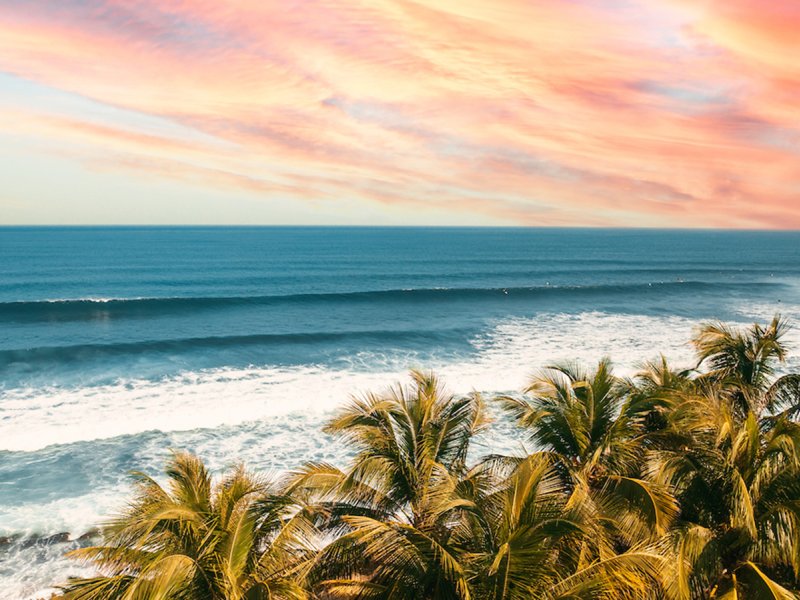The image captures a stunning tropical beach scene during what appears to be sunset. The sky is an exquisite blend of peach, orange, yellow, and hints of blue, streaked with mauve and gray, creating a mesmerizing backdrop. The deep blue ocean is largely calm, with several layers of waves, some of which are larger and appear to be tall or wide. Near the foreground, white waves wash up onto the shore. On the bottom part of the image, concentrated more on the right side, are numerous greenish-brown plants with long, thin leaves that sway leftward in the wind. Among these plants, palm trees with long fronds are prominent, adding to the tropical ambiance. The horizon is clear, with no visible land, emphasizing the vastness of the ocean and the expansive sky.